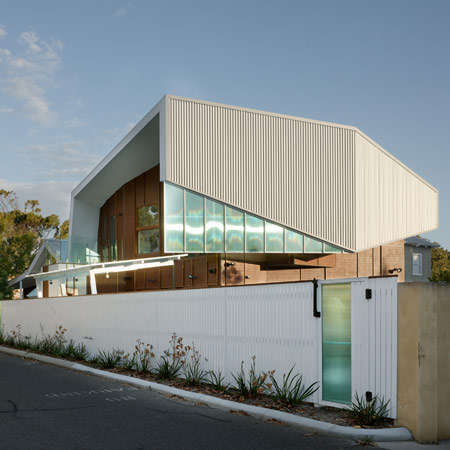The photo depicts a distinctive modern-style building located just along a paved street with a white curb. The street is bordered by a sidewalk, adorned with a variety of plants and flowers right in front of a white outer wall or gate. The modern building behind the wall contrasts with its surroundings, featuring a dark wood facade and numerous windows with a greenish tint. The structure boasts an unusual roof design that starts flat at the top and angles downward on the right side, with tan coloring. Just below the slanting roof, there is a section of glass windows that appear almost mirrored. On the left side of the image, a tree is visible against a light blue sky with a few scattered clouds. Additionally, a green door is located to the right along the wall, adding to the modern aesthetic of the building. Cracked concrete is noticeable in the lower right corner of the image, with another house partially visible in the background.